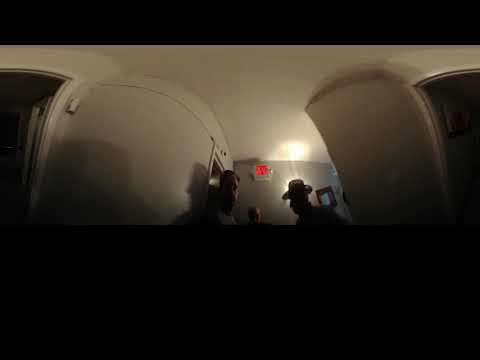In this low-resolution, heavily compressed image taken in a very dark room, two men stand prominently against white walls, illuminated by a single light behind the man on the right, who appears to be wearing a hat. Positioned almost in the center of the image, the men are nearly silhouetted due to the darkness, with only their upper halves visible from shoulders to head. The image is framed by black horizontal bars: a larger one occupying nearly three-eighths of the bottom and a thinner one at the top. To the left of the man on the left, there's a door-like box shape, and the right side of the image features another unclear square with a blue interior. There is a red exit sign beside the light source near the top right, hinting at an indoor setting, possibly a hallway or a commercial building. The curvature suggests some form of distortion, giving the impression of a warped, fisheye effect, enhancing the mysterious atmosphere of the space.